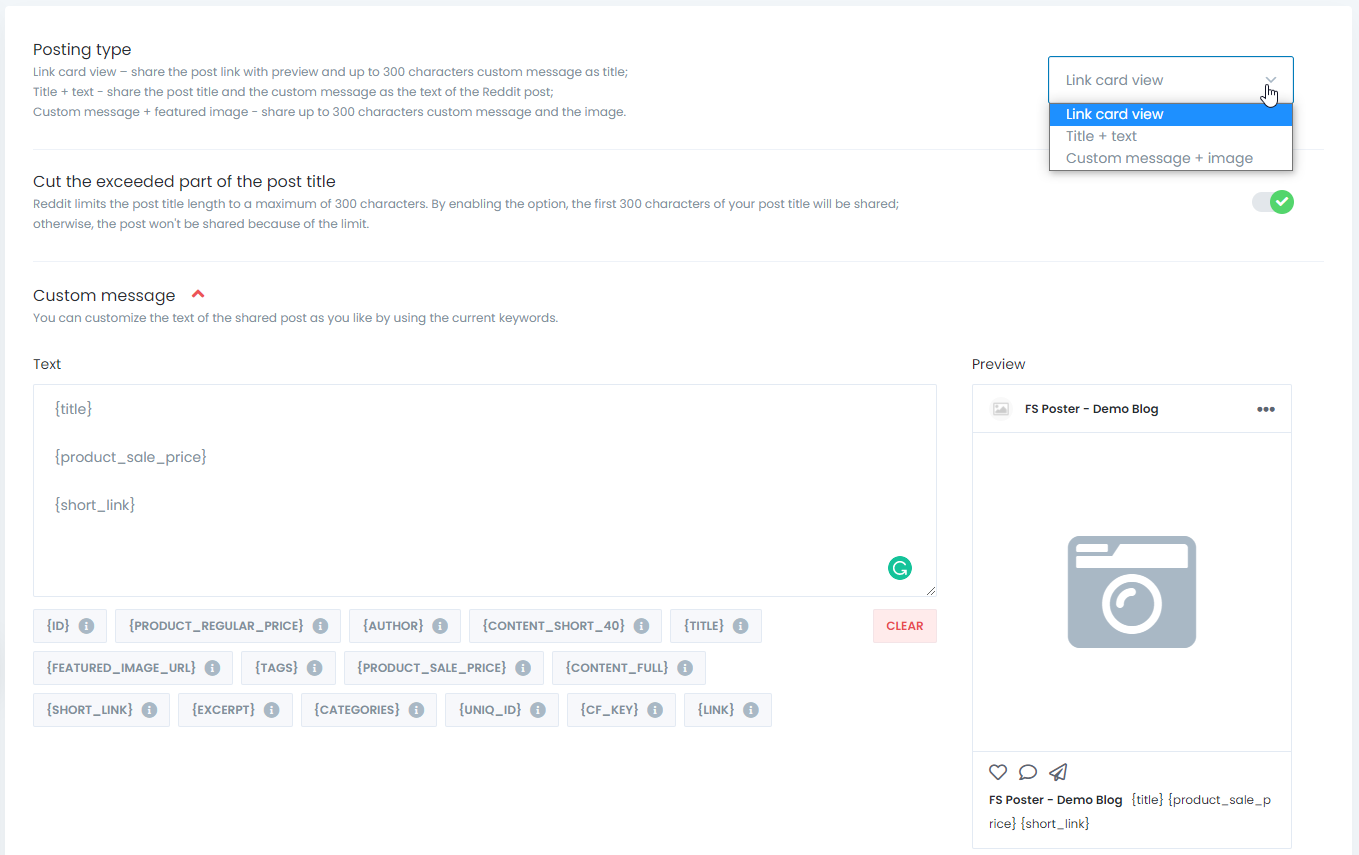**Image Description:**

The image is a screenshot of a website, predominantly featuring a white background with gray text. 

In the upper left-hand corner, several options and instructions are provided:
- "Posting Type: Link Card View"
- "Share the past link with preview and up to 300 characters custom message as the title."
- Options include "Title Plus Text" and "Share Post Past Title in the Custom Messages as the Text of the Reddit Post," among others.

A detailed breakdown is given for how to configure the post, including:
- "Custom Message Plus Featured Image: Share up to 300 characters custom message and the image on the right-hand side."
- "Link Card View: Title Plus Text or Custom Message Plus Image."
- Notation that "Reddit limits the post title length to a maximum of 300 characters. By enabling the option, the first 300 characters of the post title will be shared; otherwise, the post won't be shared due to the limit."

Additional customizable options are provided:
- A prompt to "Custom Message: Customize the text of the shared post as you like by using the current keywords."
- Examples of keywords include "[Title], [Product Sale Price], [Short-Link]."

Below this section, a preview of the content is shown with the label "This is FS post or demo blog" alongside a camera icon image.

At the bottom of the page, various metadata tags enclosed in brackets are listed:
- [ID]
- [Product Regular Price]
- [Author]
- [Content Short Title]
- [Featured Image URL]
- [Tags]
- [Product Sale Price]
- [Content Full], [Short-Link], [Excerpt]
- [Categories]
- [Unique ID]
- [CF Key]
- [Link]

This screenshot provides a comprehensive guide on how to format and customize a post for sharing, specifically tailored for Reddit.